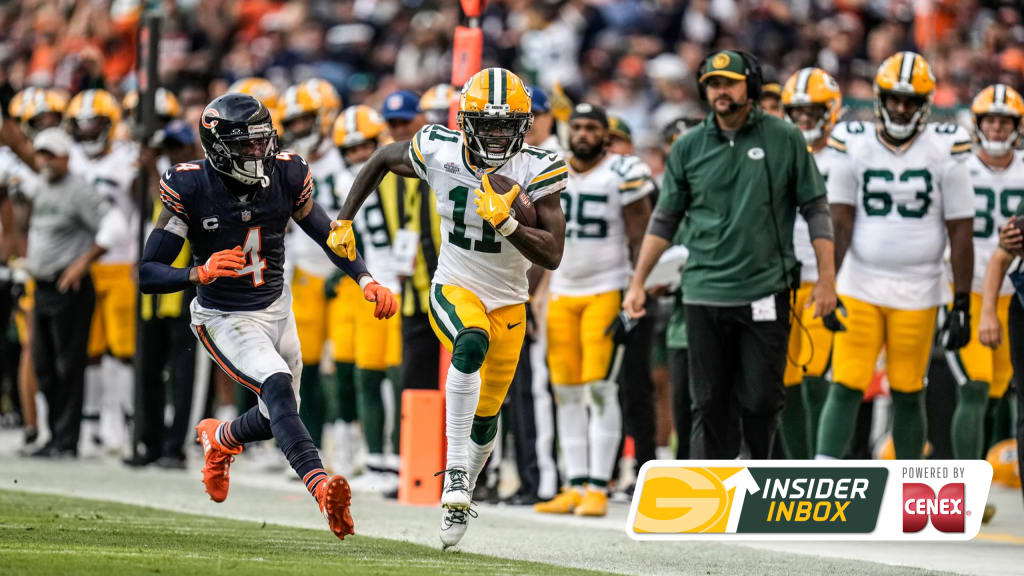In this detailed photograph from an NFL football game, player number 11 from the Green Bay Packers is captured running with the ball. He is wearing a yellow, white, and black helmet, a white jersey with green lettering and yellow accents, yellow pants with green and white striping, and white socks. He is being pursued by player number four from the Chicago Bears, who is dressed in a navy blue helmet, navy blue jersey, white pants, and navy blue socks. Along the sideline, players and coaching staff in various team attire watch the action unfold, with a blurred crowd visible in the background. A referee or coach, identifiable by his green golf shirt, green and yellow cap, and black pants, stands prominently in the bottom right. An overlay in the lower right corner reads "Insider Box powered by Cenex" in white text on a red background, adding a digital element to the scene.